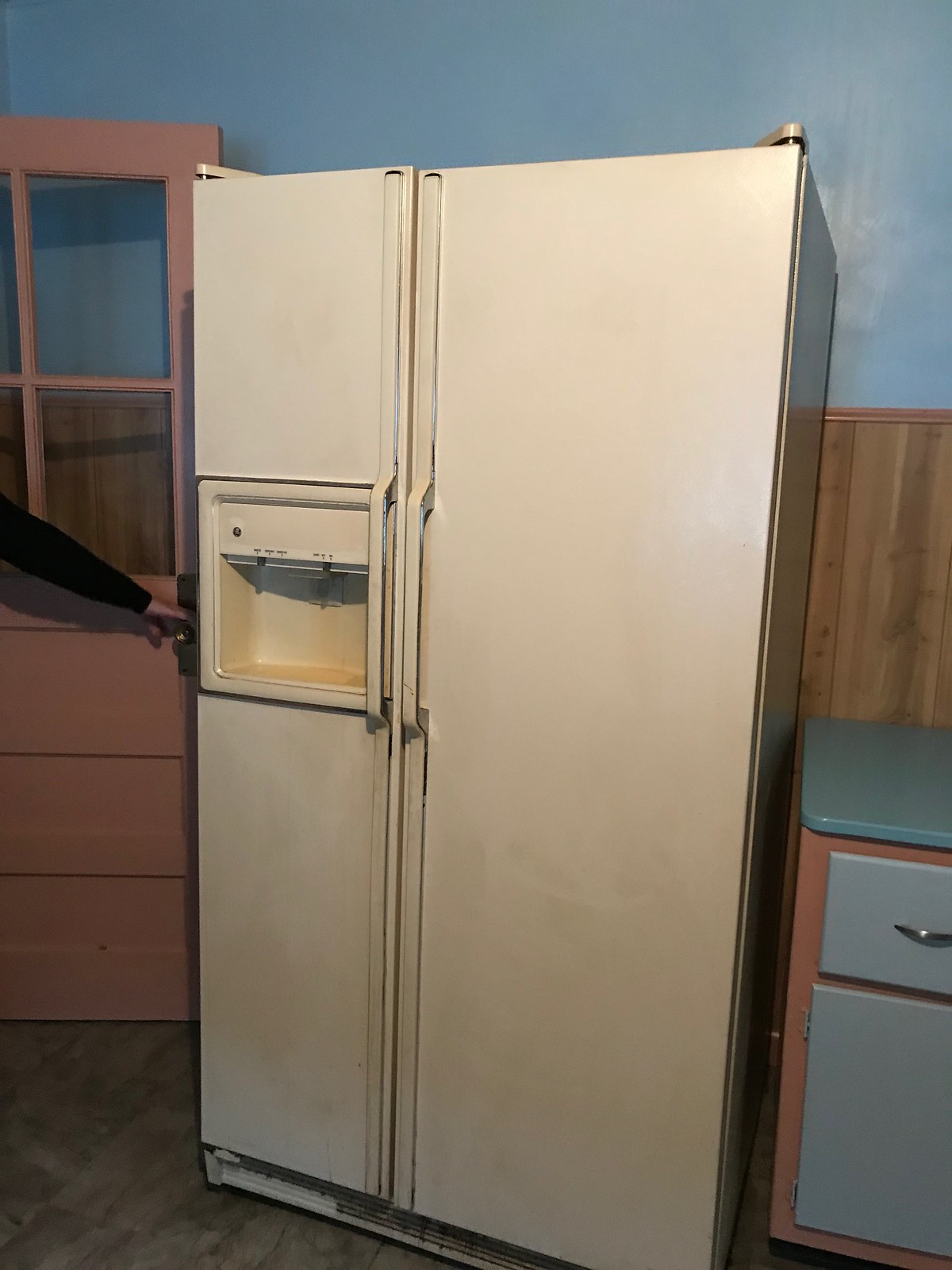The image captures a well-worn, double-door refrigerator from the 1990s or early 2000s, situated in the center of a kitchen scene. The left-hand side of the refrigerator, which is thinner than the right, features old-style ice and water dispensers. The once white surface of the refrigerator has aged, showing brown discoloration, particularly around the dispenser area, and yellowing over time. A moldy vent can be seen at the bottom. The door handle is positioned in the middle, on the skinnier, off-white left section. The background showcases a mix of blue and pink paneling with wood, and a hand in a black sleeve is visible on the left, holding a doorknob. Other kitchen details include light blue countertops, silver-handled cabinets, and weathered surfaces, reflecting the overall aged and worn condition of the space.